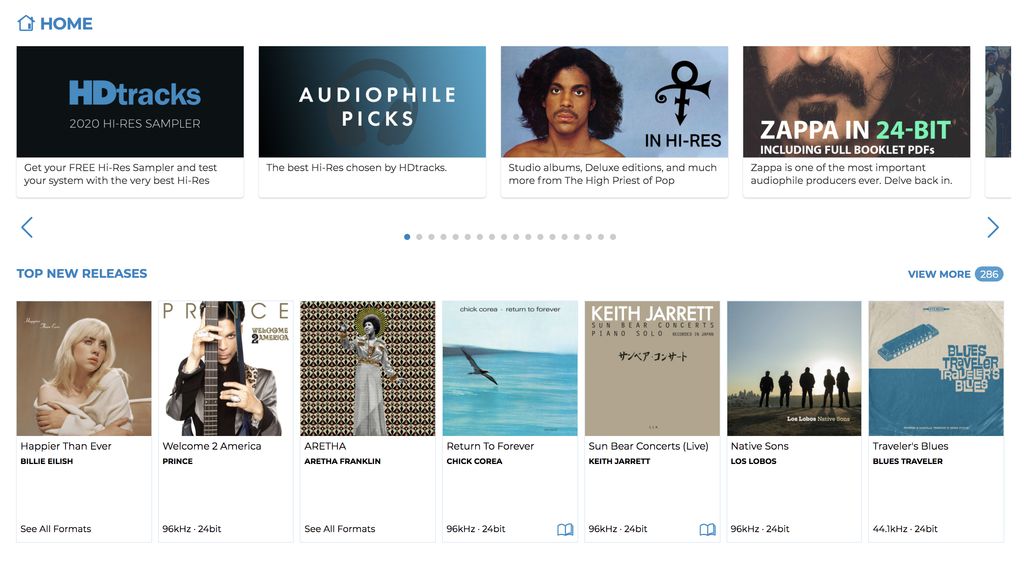This is the home screen of a music streaming platform showcasing the top new releases. Prominently displayed is Billie Eilish's album "Happier Than Ever," featuring a cover image of her wearing an off-the-shoulder white coat. She stands against a beige background, her platinum blonde hair falling to her shoulders as she gazes contemplatively to the side. Also highlighted is Prince's "Welcome 2 America," with a cover showing Prince holding a guitar such that it obscures half of his face, his hands gripping the fretboard and fingerboard. Aretha Franklin's album "Aretha" is celebrated with a nostalgic image of the iconic singer sporting an afro and wearing a long white gown, set against a patterned backdrop. Another prominent feature is Chick Corea's "Return to Forever," whose album cover depicts a serene ocean scene with a large bird skimming the water. Lastly, Keith Jarrett's "Sun Bear Concerts (Live)" is listed, though its cover image is not described in detail.